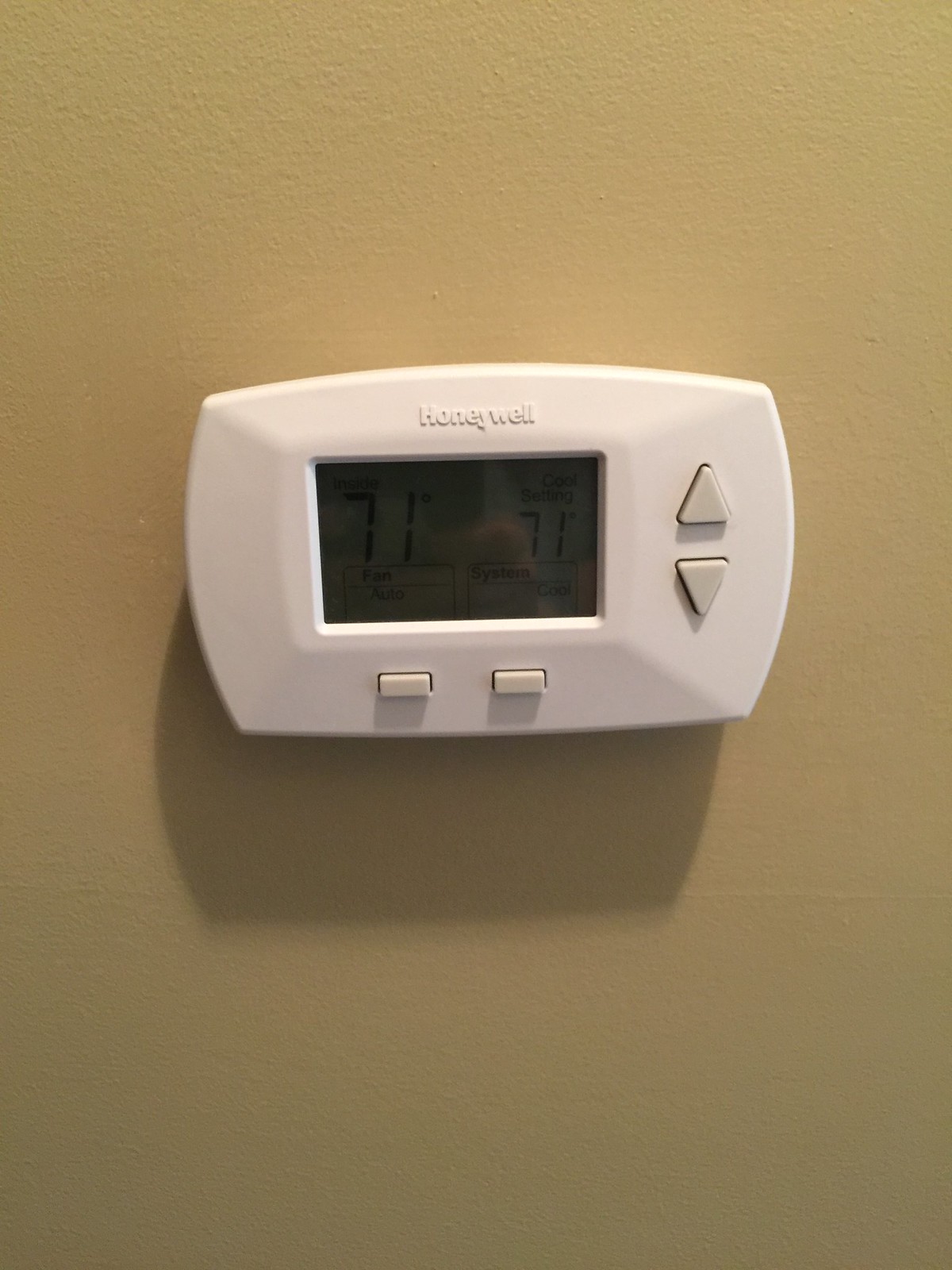In this portrait-oriented photograph, the focus is on a Honeywell temperature controller mounted against a dark tan wall. The device is white and rectangular, featuring a set of controls and a digital screen. On the right side, there are up and down arrows for adjusting the temperature. Below these arrows, at the bottom of the controller, two additional buttons are present. The digital display, although dimly lit, shows a temperature reading of 71 degrees Fahrenheit on the left side and indicates that the system is set to 'Cool' at 71 degrees on the right. Below the primary temperature display, the words 'Fan' and 'Systems' are faintly visible. The Honeywell logo, subtly embossed at the top of the controller, stands out against the matching plastic surface.